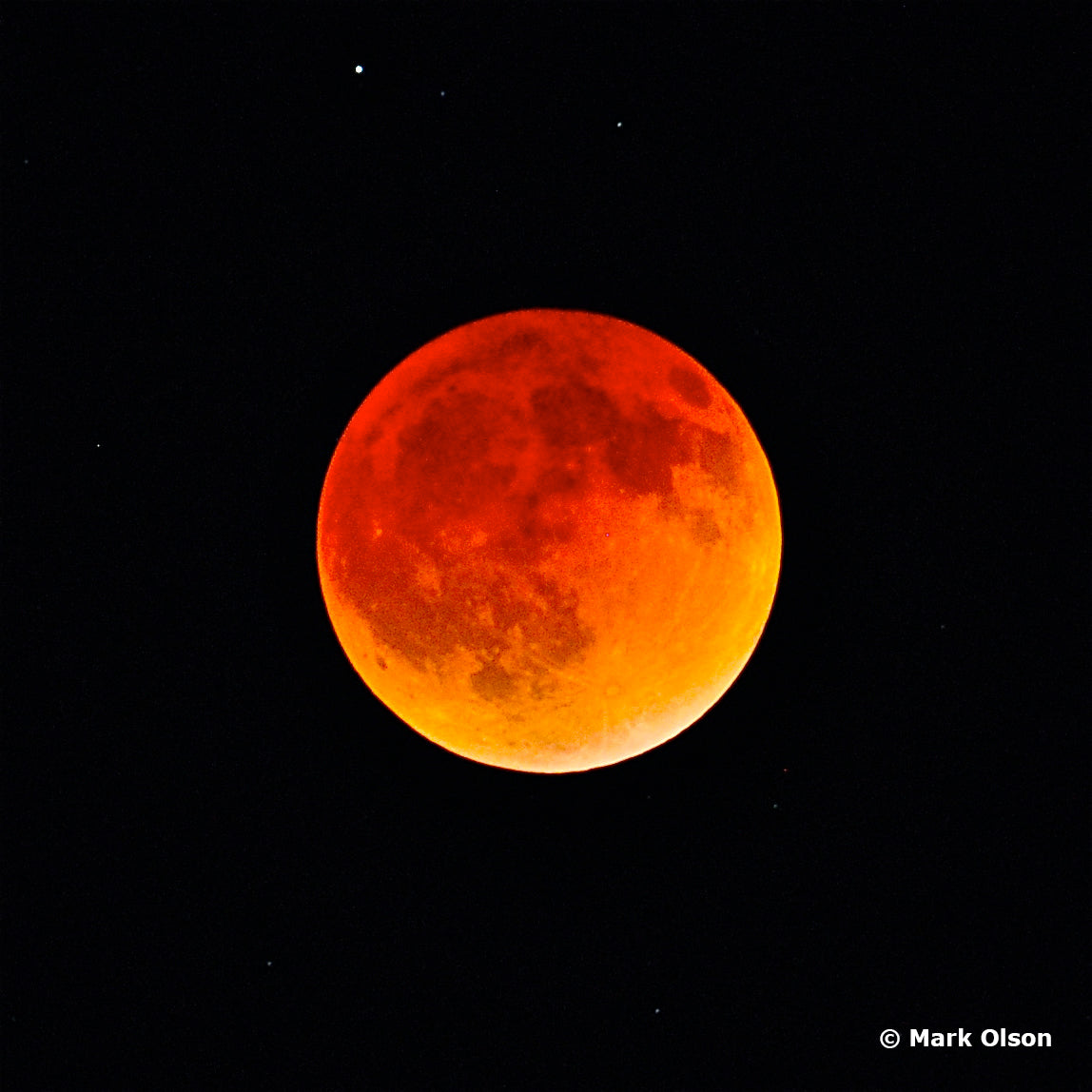The image features a perfectly square frame with a predominantly black background, punctuated by three white dots of varying sizes at the top center, representing stars. Central to the image is a vividly colored depiction, likely of the moon, transitioning from red at the top to orange and then yellow towards the bottom. The texture within this celestial body seems to suggest an artistic rendering, possibly a computer-generated graphic, rather than an actual photograph. In the lower right-hand corner, the white copyright symbol "©" is followed by the name "Mark Olsen" in white font. There are no additional elements, people, text, or colors, making the focus solely on the striking, gradient-hued moon and the subtle star details against the stark black backdrop.